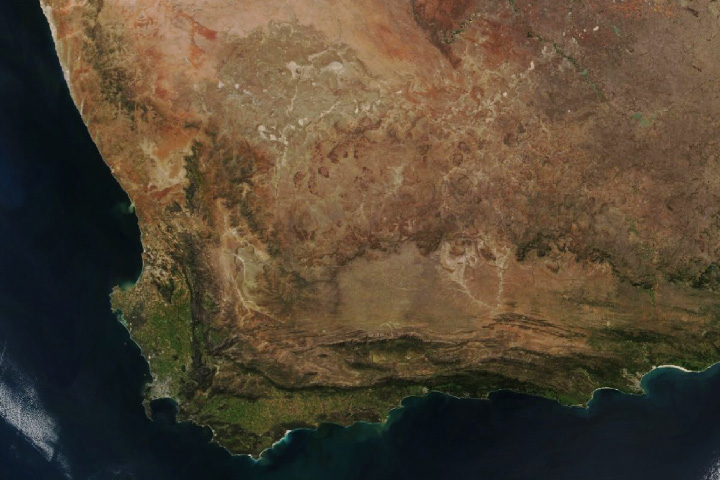This aerial or satellite image, seemingly taken from a considerable altitude, possibly space, presents a striking view of an island surrounded by a vast, dark expanse of ocean. The majority of the image depicts the island, which has a distinct green area at the lower part, transitioning to darker brown hues towards the island's interior, suggesting varied terrain possibly including mountainous regions. Along the lower left, upper left, and bottom right corners, the dark ocean dominates, with visible white streaks and foam indicating waves breaking against the shore. The shorelines are particularly noticeable where the water meets the island, framed by white foamy waves. The image's zoomed-out perspective highlights the island's uneven, natural topography, giving it an almost planetary appearance, with green coastal regions fading into rugged, brown inland areas.